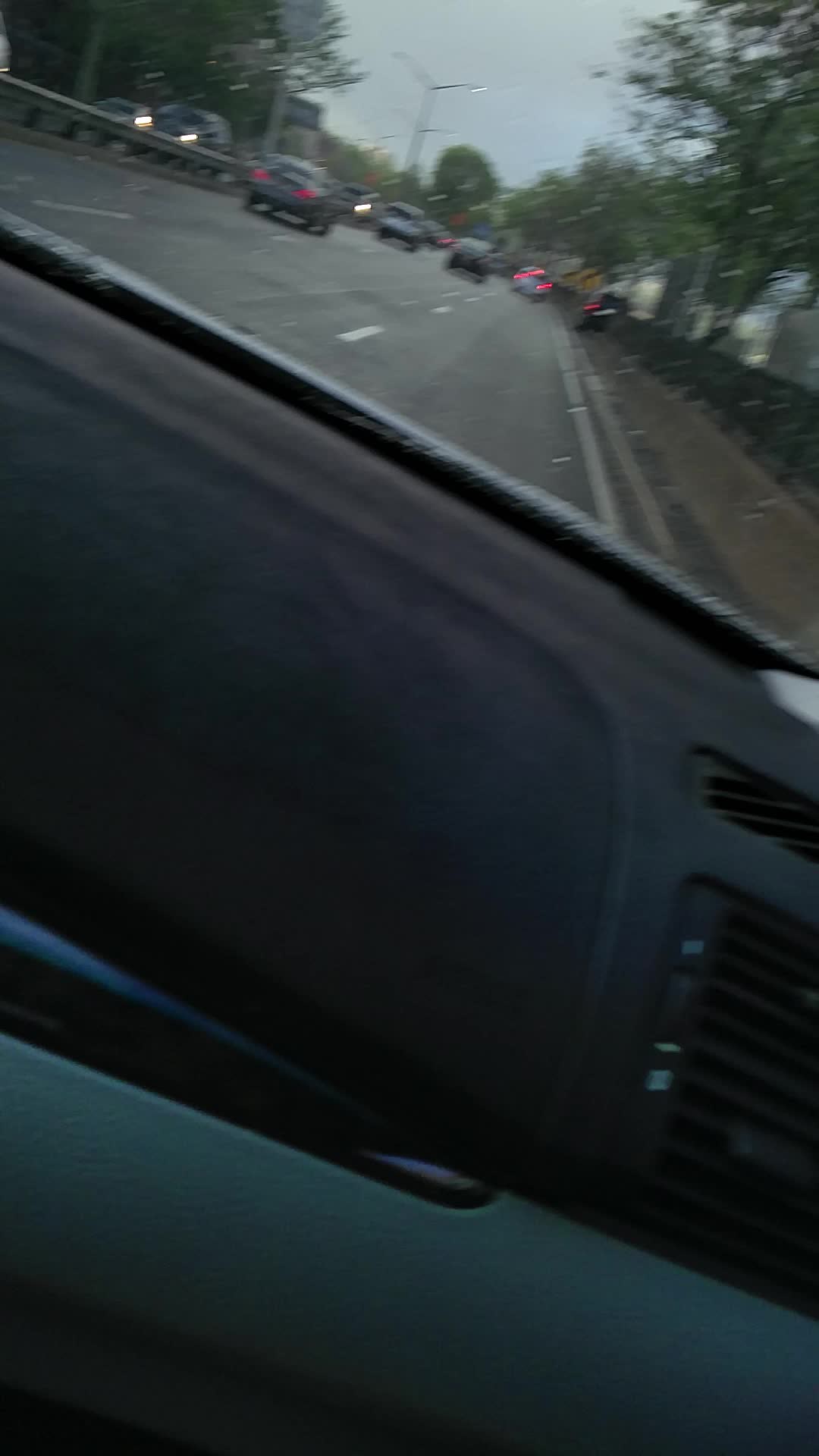The photograph presents a driver's or passenger's perspective within a vehicle, showcasing a dashboard that transitions from a dark grey at the top to a lighter grey below. Prominently visible are black air vents, one positioned to the right and another towards the upper section of the dashboard. The front windshield provides a clear view of a grey asphalt road delineated into three lanes by white dashed lines, along which several vehicles are traveling. The sky appears to be overcast with a light grey hue, suggesting an overcast day. 

On the right side of the road, a dark grey railing rises from a similarly grey cement base, while traffic is seen moving in the opposite direction on the left side. Further accentuating the scene, there are green trees lining both sides of the road, contributing to a natural roadside ambiance. Streetlights can also be seen in the distance, characterized by light fixtures arranged in a Y formation. Additional details include a car ahead with illuminated red taillights, highlighting the ongoing traffic conditions. The setting suggests a bustling yet orderly roadway environment, potentially reminiscent of a major arterial route like Lakeshore Drive.